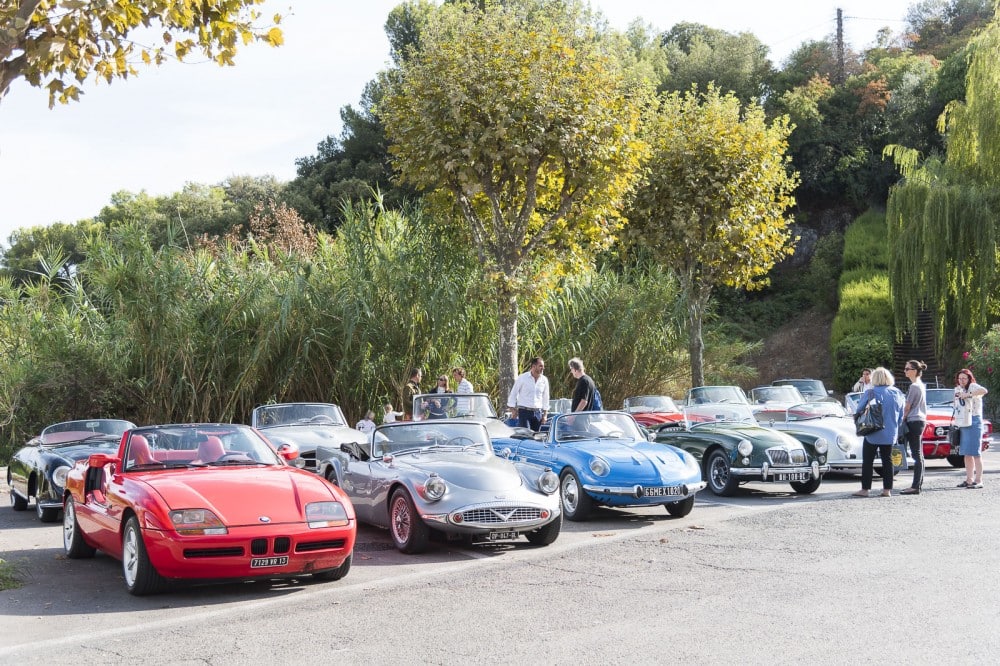The image depicts an outdoor classic car show with a neat arrangement of vintage convertibles parked diagonally in two rows. The scene unfolds on a light gray cement surface, hinting at an expansive open area. The showcased cars, displaying European license plates and all with their tops down, include a variety of colors and models: a distinctive red convertible at the forefront that might resemble a BMW, a silver car reminiscent of the classic Aston Martin seen in old James Bond films, a blue car, a dark green car, and another silver car.

In the background, lush, diverse greenery frames the event, with tall lime green trees standing against a pale sky and green bushes forming a natural backdrop. Various people, including a group of middle-aged men along with three women on the right—one of whom carries a black purse—wander among the cars, engaged in conversation and admiration. Additionally, a staircase can be seen behind the cars, further indicating the park's expansive setting. This scene captures the essence of a lively classic car meetup outside the United States, filled with enthusiasts appreciating the timeless elegance of these old models.